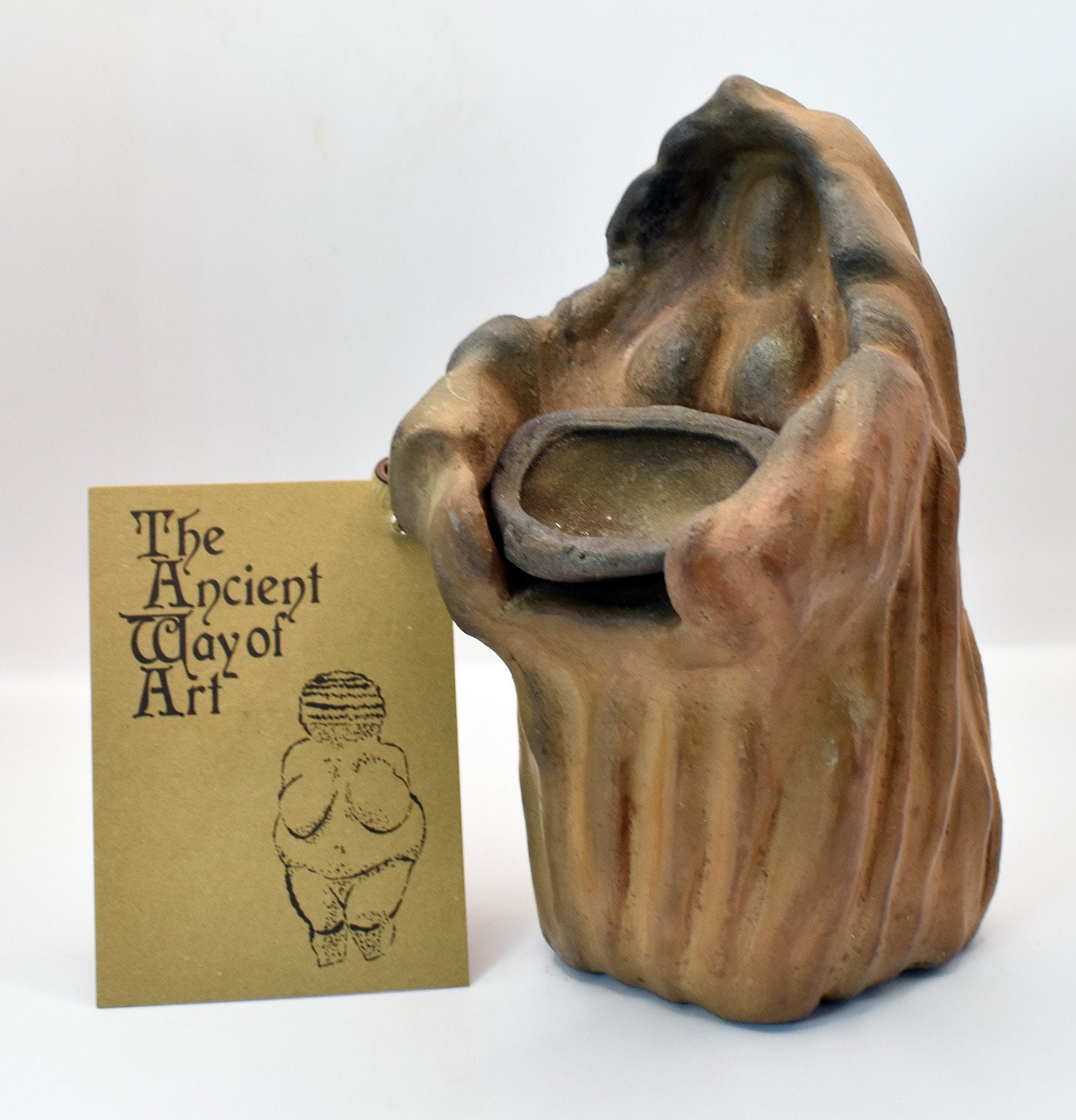The photograph features a distinctive art display set against a gradient gray background, lighter at the bottom and darker at the top. On the lower left of the image is a greenish-brown card with an old-fashioned, black-font title reading "The Ancient Way of Art." Below the title, a charcoal sketch illustrates an ancient, rotund feminine figure with prominent breasts, lacking detailed facial features, arms, or feet.

To the right of the card stands a primitive clay or stone sculpture. The sculpture is predominantly brown with hints of black tinge on the edge of its robe. It features a robust figure draped in a cloak, with only the outline of the face and arms distinguishable. Held within the folds of the cloak is a small bowl or dish, colored to match the rest of the monochromatic statue. The base of the sculpture is rectangular, leading up to the detailed upper body that mirrors the form described in the sketch on the card. The overall composition highlights the ancient and primitive essence of the artwork.